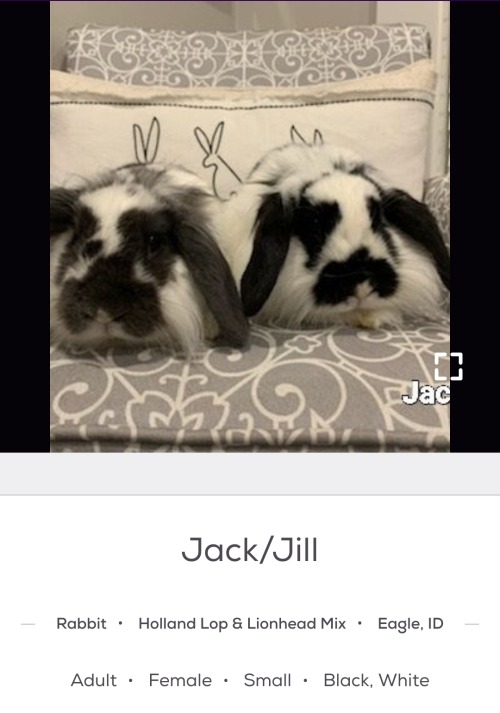In the image, there are two extremely fluffy bunnies with a mix of white, black, and grey fur. One bunny has notable black ears. They are resting on grey bedsheets adorned with white lines. In the bottom right corner, a portion of the image is occupied by what appears to be a black-toed rabbit named Jack or Joe, who is a mix between a Holland Lop and a Lionhead breed. Both bunnies are adult females. The background of the image is grey, providing a neutral backdrop that highlights the bunnies' fur textures and colors.